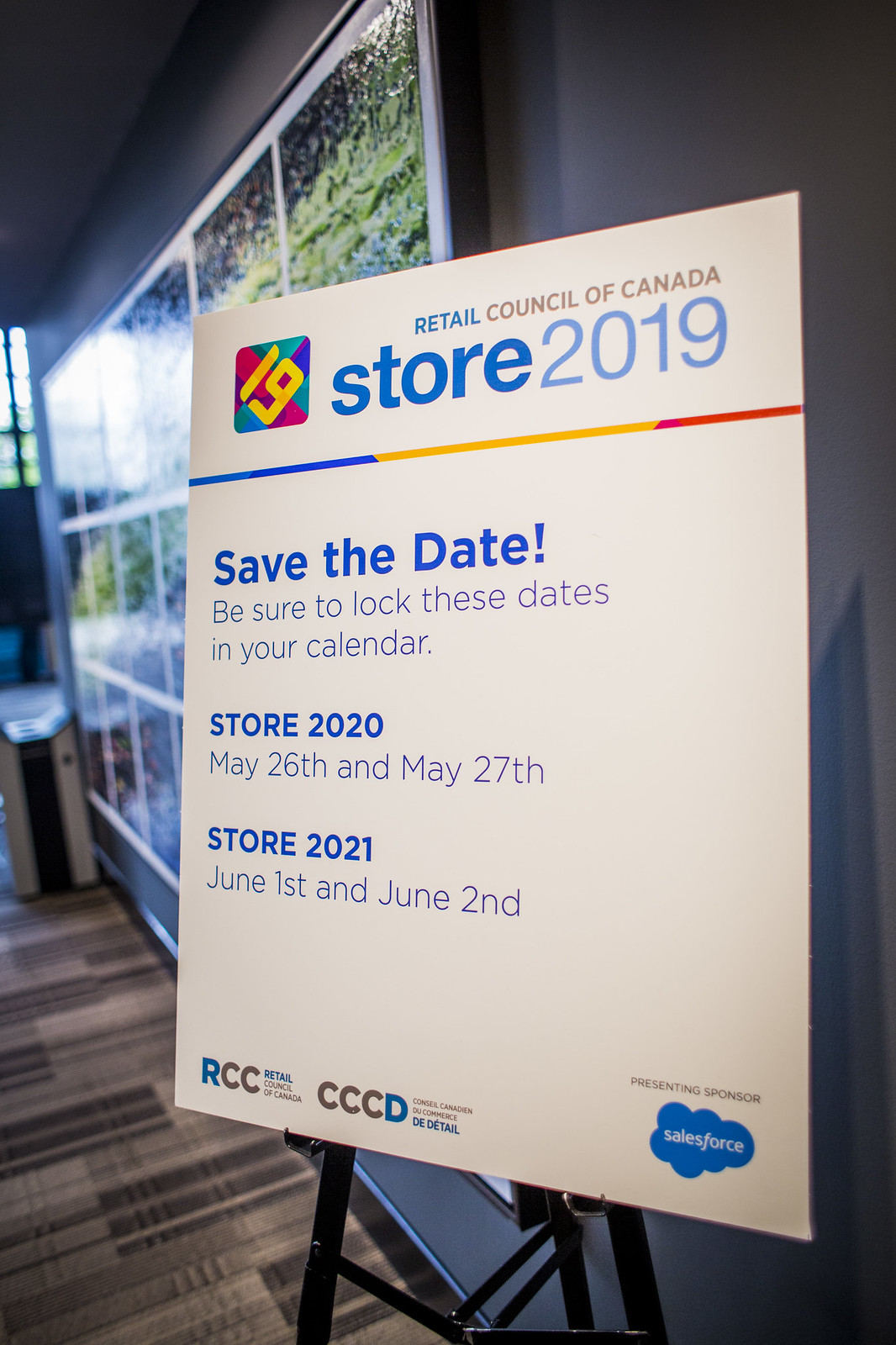The image showcases a black easel or tripod stand displaying a detailed event poster. At the top of the poster, in blue text, it reads "Retail Council of Canada" with "Council of Canada" specifically highlighted in brown. The colorful logo prominently features the number "19" in yellow, set within a rounded square that has green, purple, and pink elements. Above this logo, it says "Store 2019" in blue. A multicolored stripe runs across the poster, starting blue, transitioning to yellow in the middle, and ending in red.

The main body of the poster urges readers to "Save the Date," specifying dates for upcoming events: "Store 2020" on May 26th and 27th, and "Store 2021" on June 1st and 2nd. The bottom right corner features the Salesforce logo within a blue cloud, identifying them as the Presenting Sponsor. Further logos at the bottom include RCC for Retail Council of Canada and CCCD, which stands for the Canadian Chamber of Commerce.

The setting appears to be indoors, with a large portrait and a striped gray and black floor visible in the background. Adding to the ambiance, there are various pieces of art and tiled decorations in the vicinity, as well as a tan and black striped carpet on the floor.